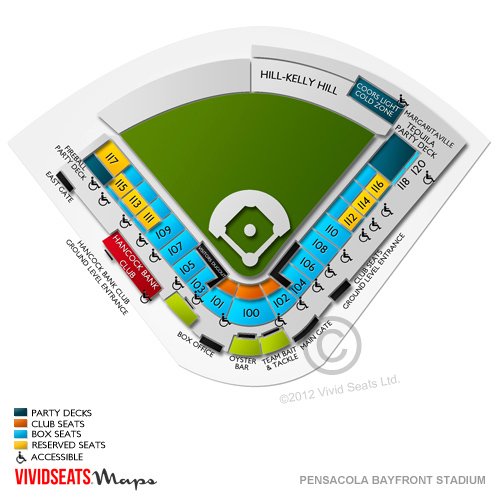This is a detailed seating chart screenshot from Vivid Seats Maps showcasing the layout of Pensacola Bayfront Stadium, an amphitheater-shaped venue resembling an inverted triangle with rounded corners. The map highlights seating arrangements and various sections designed for a baseball field setup.

In the image, the sections closest to the field are marked in blue, specifically labeled as the 100 section, indicating prime seating areas for optimal viewing. Notably, reserved seats are highlighted in yellow: on the left side, they encompass sections 111, 113, 115, and 117; on the right side, they include sections 112, 114, and 116.

Distinctive areas such as the Tequila Party Deck, denoted in dark green, lie behind section 116, catering to attendees who prefer a lively atmosphere. On the opposite side, a smaller Fireball Party Deck is located, adding to the venue’s festive options. Within the 100 section, numerous wheelchair-accessible seats ensure inclusivity.

The Hancock Bank Club offers exclusive club seating at the upper left of the seating area, while box office seats, highlighted in proximity to the bottom center, provide premium viewing options.

A legend at the bottom left of the map clarifies the color coding: dark green indicates party decks, orange signifies club seats, blue represents box seats, yellow denotes reserved seats, and a wheelchair icon marks accessible seating areas. Below the legend, "Vivid Seats" is written in red, followed by "Maps" in black. At the bottom right corner, "Pensacola Bayfront Stadium" is inscribed in gray text. Additionally, a watermark reads "© 2012 Vivid Seats LTD," ensuring the authenticity of the map.